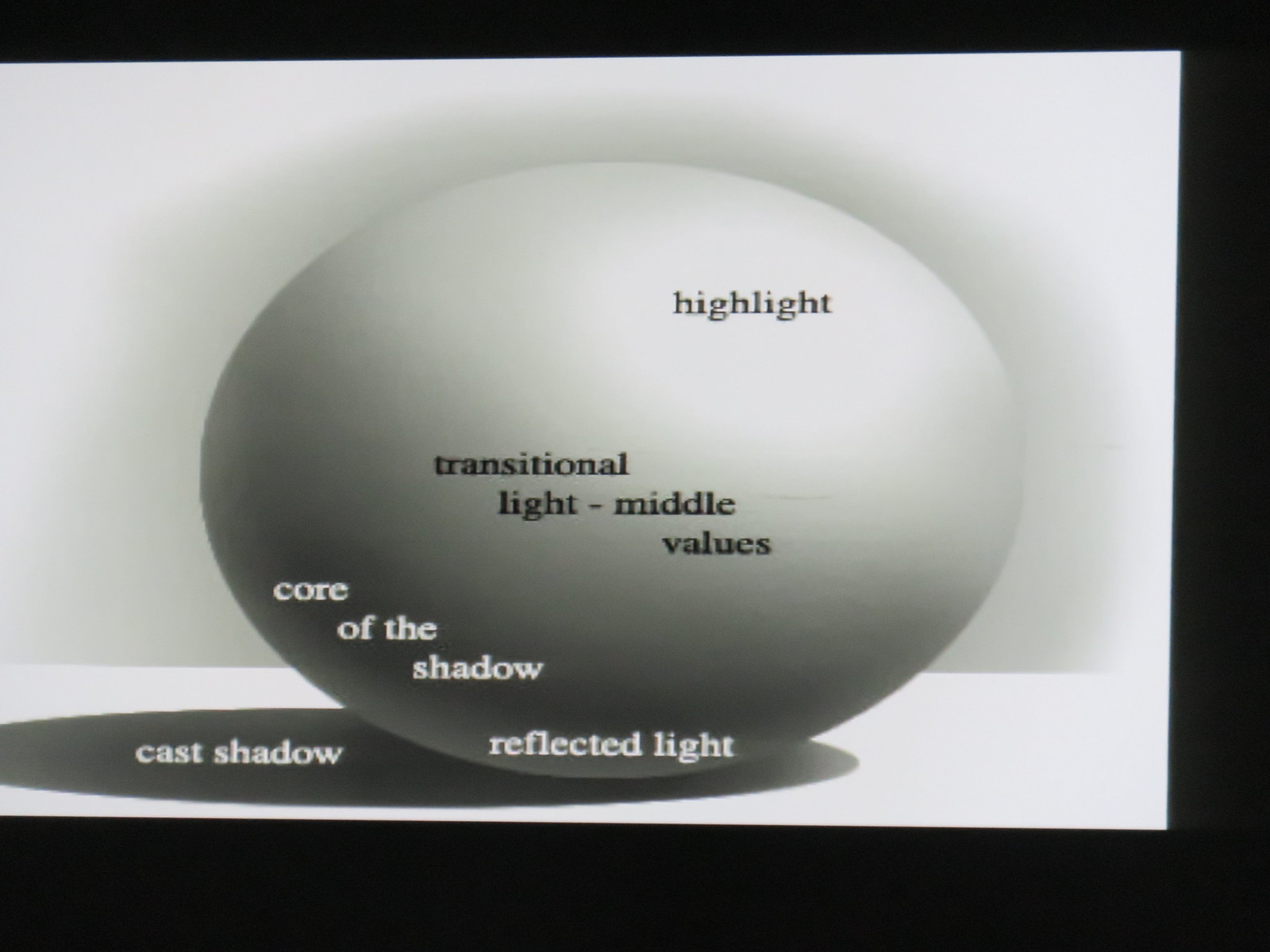The image features a horizontally oriented, egg-like sphere set against a white background with a black border on the top, right, and bottom edges. The left side of the border is missing. The sphere casts a subtle gray shadow, creating the appearance of a gray spray paint effect behind it. The image serves as an instructional art piece, labeling different forms of shading on the object. 

On the top right of the sphere, the term "highlight" is written in small black letters. In the center, "transitional light, middle values" is displayed in prominent black text. The left side of the sphere reads "core of the shadow, reflected light" in white font. At the bottom left, within the dark shadow, the term "cast shadow" is labeled in white letters. This detailed diagram effectively illustrates the different aspects of light and shadow, guiding viewers through various shading techniques.